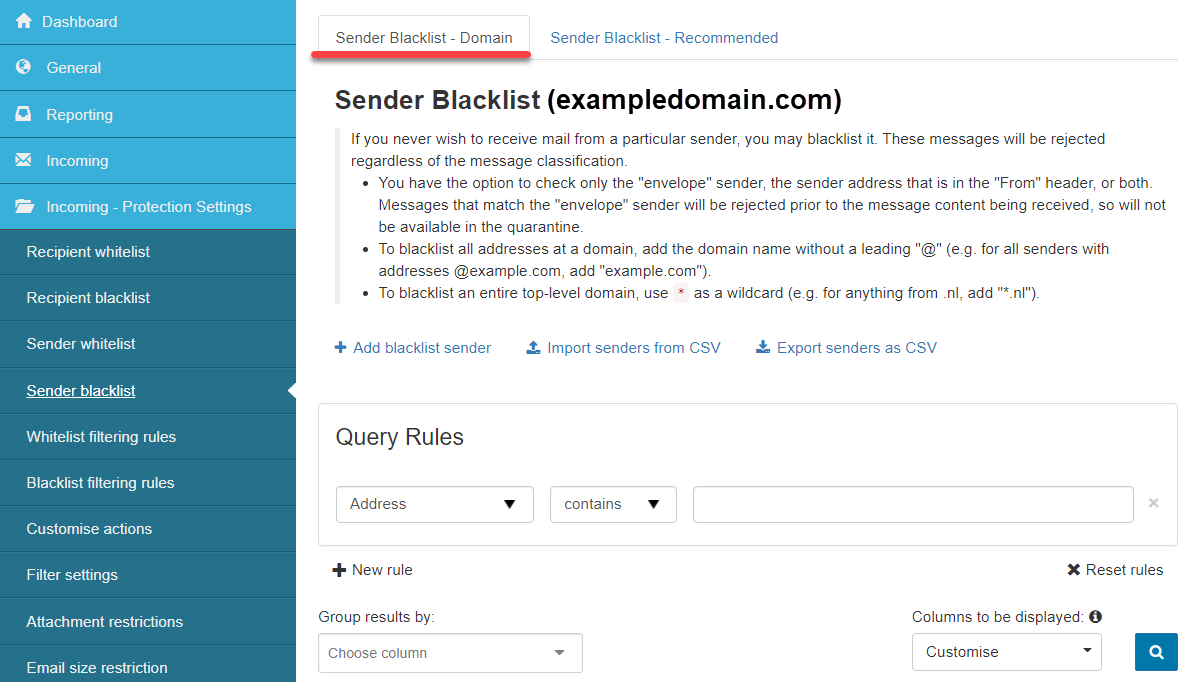**Detailed Caption:**
The image showcases an interface with a vertical site menu on the left side. The menu is divided with a lighter blue at the top section and a darker blue at the bottom section, with the text in white. The menu items listed include: Dashboard, General, Reporting, Incoming, and Incoming Protection, each using a light blue background, followed by Recipient White List, Recipient Black List, Sender White List, Sender Black List, White List Filtering Rules, Black List Filtering Rules, Customize Action, Filtering Settings, Attachment Restriction, and Email Size Restriction, which all have a dark blue background.

On the right side of the interface, there is a highlighted text "Send Black List Domain," underlined in red, and beside it, the text "Send Black List Recommended." Below this, there's informational content stating: "Send a Black List Example Domain.com. If you never wish to receive mail from a particular sender, you may blacklist it. Messages will be rejected regardless of the message classification. You have the option to check only the envelope sender. The sender address that is in form header or both messages that match envelope sender will be rejected prior to the message content being received, so it will not be available in the quarantine. To blacklist all addresses, add a domain name without a leading e.g., for all senders with the address, add example.com. To blacklist an entire top-level domain, use '*' as a wildcard."

At the bottom of the image, there are three blue buttons labeled: Add Blacklist Sender, Import Sender CSV, and Export Sender CSV. Additionally, there are sections for Query Rules, Address, Content, an empty spacebar, and a Reset Rule button. The bottom part of the interface also contains options for Group Result By and Choose Column. On the bottom right, it indicates "Column to be Displayed," a Customize option, and a Blue Search Box.